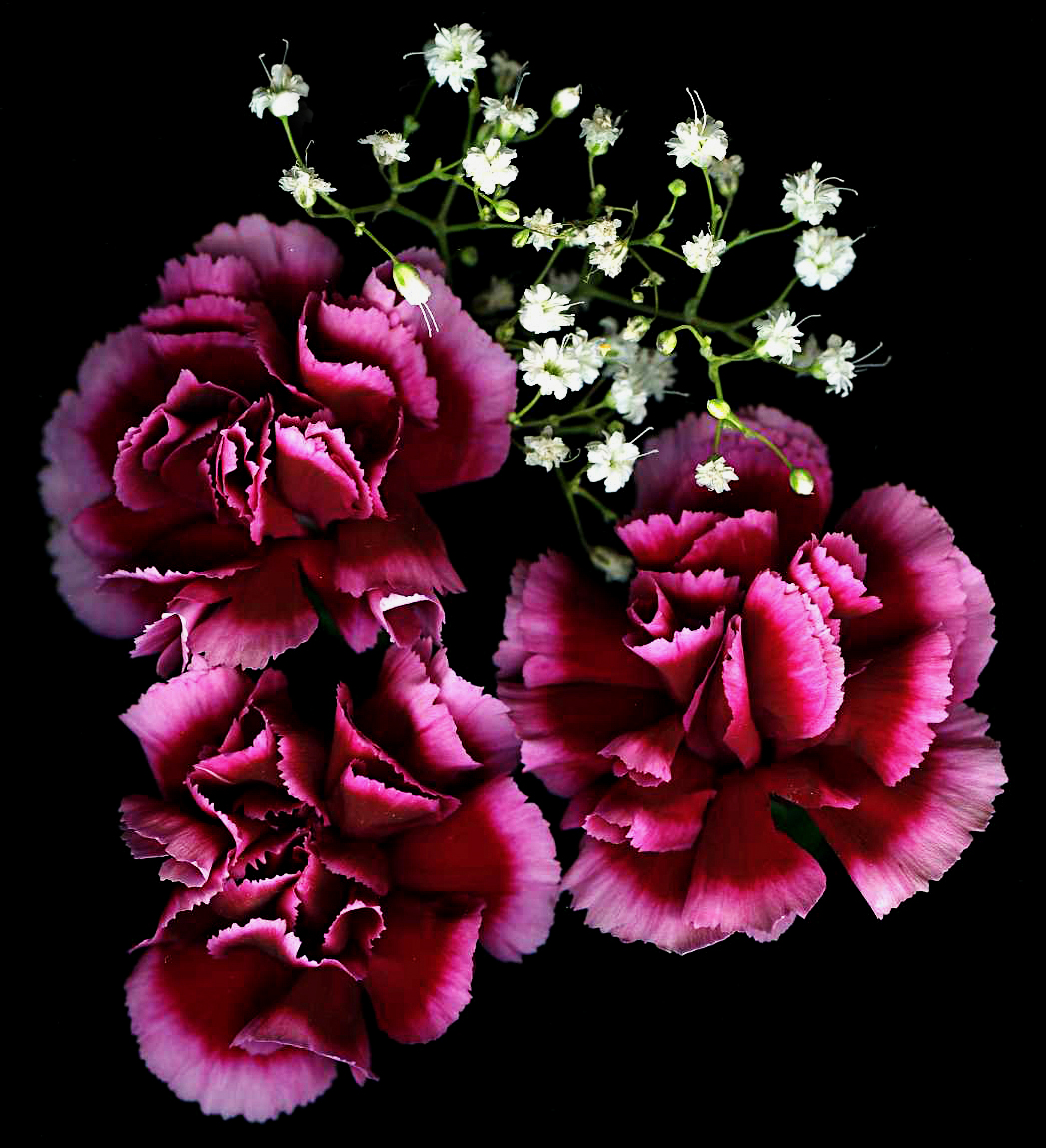This image features a high-quality, detailed drawing of three large roses set against a solid black background. The roses, which dominate the center and lower portions of the image, are depicted with a gradient of dark pink transitioning to light pink and almost white at the scalloped edges. Shadows add depth to the densely layered petals, enhancing their realistic appearance. The roses are arranged in a triangular formation, with one at the bottom left, one at the right, and one looking slightly off to the left. Above these prominent roses, a cluster of smaller white flowers emerges from thin green stems, creating a delicate contrast with the bold pink hues below. These tiny white flowers have soft petals with two lines extending from their centers, adding intricate detail to the composition. The background remains pitch black, providing a stark and striking contrast that makes the vibrant colors of the flowers stand out.